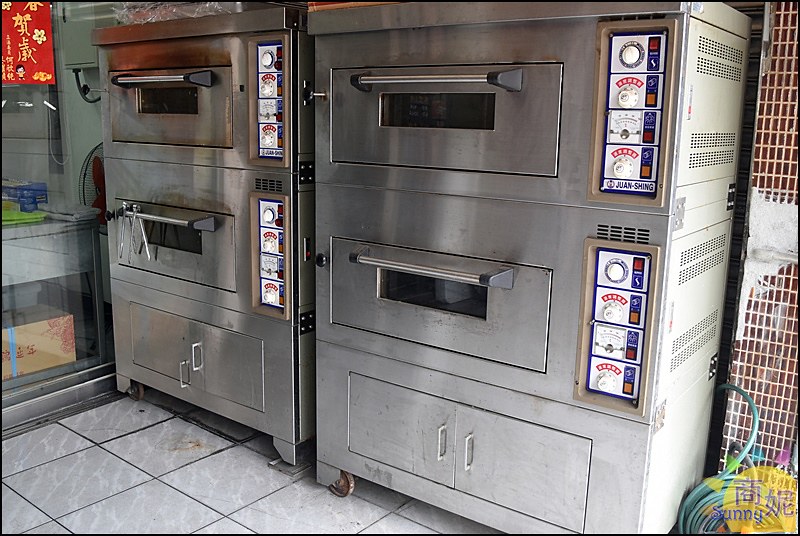The digital photograph showcases a commercial kitchen likely within a Chinese takeaway, distinguished by Asian script (Chinese or Japanese characters) on a small red flag with tan lettering and a white flower, positioned in the upper right corner. Dominating the scene, four large stainless steel ovens are arranged in a 2x2 configuration against a slightly sloping wall that recedes into the top left side of the image. Each oven unit comprises two stacked ovens, each featuring a black rectangular window and large horizontal handles with black end pieces. On the bottom left oven, stainless steel tongs hang over the handle. Each unit is equipped with four dials and rows of ventilation slits on the right.

Notably, the ovens rest on a tiled floor adorned with black grout lines between white marbled tiles, which are somewhat dirty and littered with brown crumbs and detritus. The wall to the ovens' right is adorned with red acrylic pieces and white grout, further reinforcing the kitchen's functional aesthetic. In the bottom right corner, a green garden hose is visible, and additional Asian script alongside the word "sunny" in blue print can be discerned. The image also notes that the left handle on the rightmost oven appears broken, hanging downwards. Lastly, the ovens are depicted on casters, suggesting they can be moved as needed within the space.